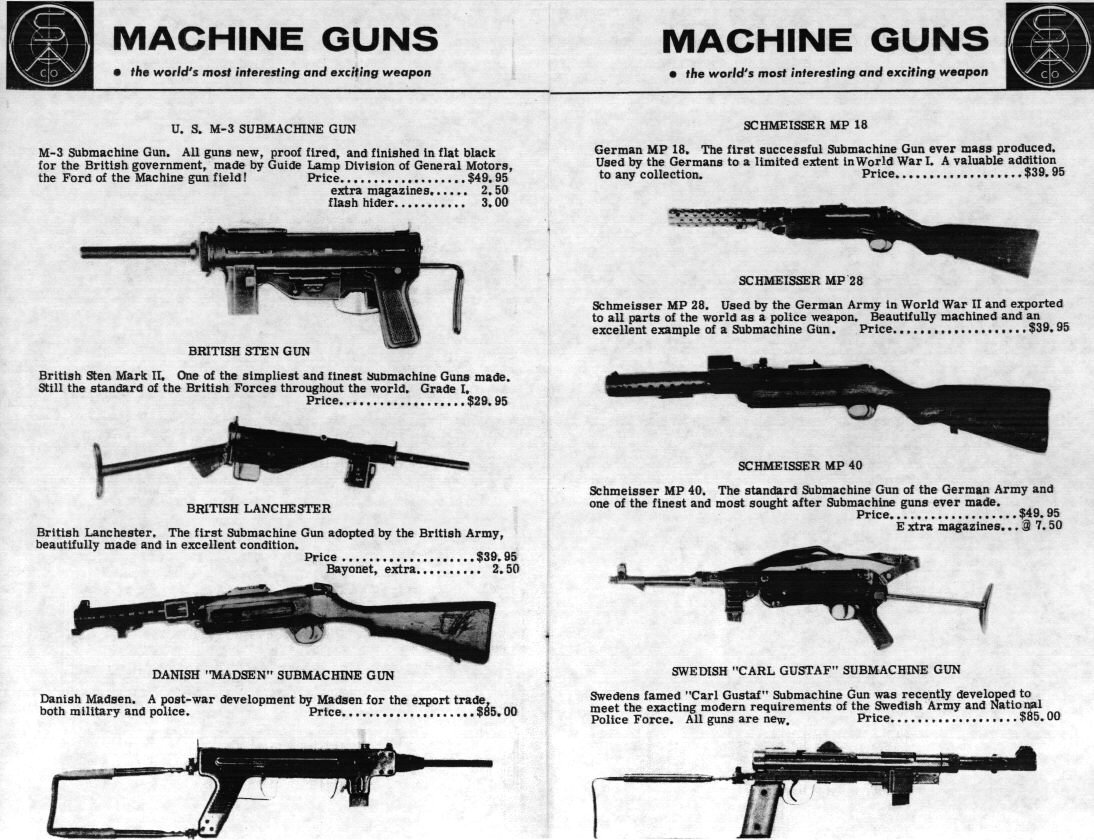The image appears to be a photocopy of a vintage two-page magazine spread from a gun-related publication. The title at the top of both pages reads, "Machine Guns: The World's Most Interesting and Exciting Weapons." The spread showcases eight different types of machine guns, with all images rendered in black and white. The featured firearms include the US M3 submachine gun, the British Sten gun, the British Lanchester, the Danish Madsen submachine gun, the Schmeisser MP18, the Schmeisser MP28, the Schmeisser MP40, and the Swedish Carl Gustaf submachine gun. Each gun is accompanied by a price and, in some cases, additional pricing details for accessories such as extra magazines or bayonets. The overall aesthetic and presentation suggest this is an old sales advertisement, with a visible book seam running down the middle of the spread. The guns are presented in various shapes, some resembling classic machine guns, while others have a rifle or shotgun-like appearance.